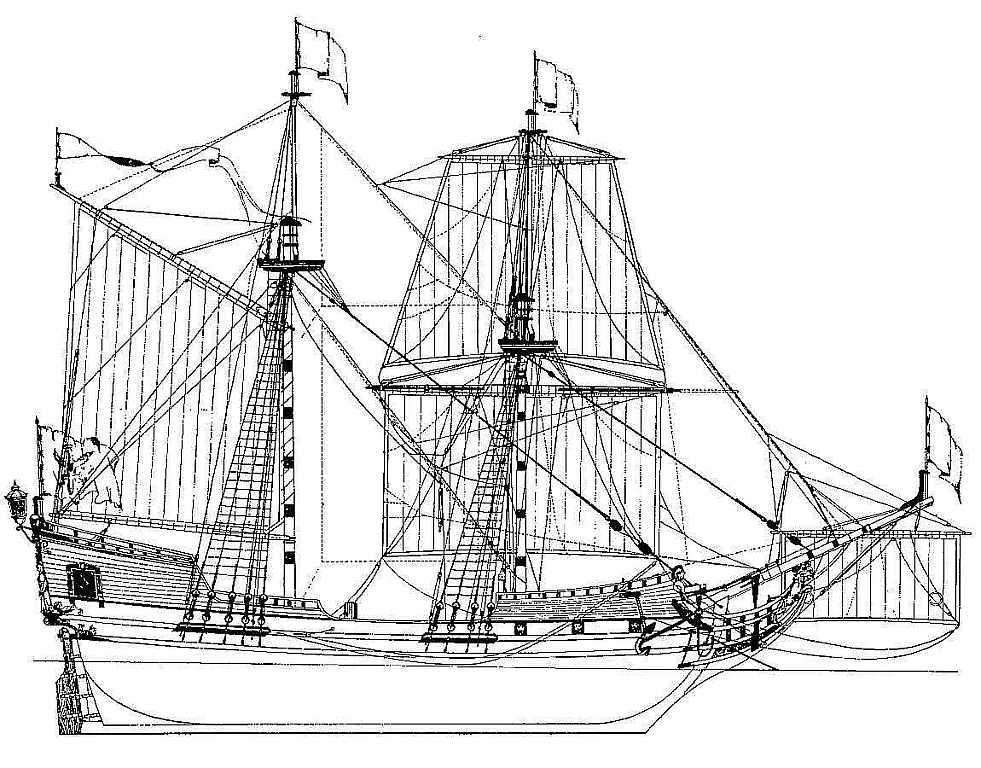This detailed black-and-white hand-drawn illustration depicts a side profile of an old galleon sailing ship, commonly used for long sea voyages and exploration. The ship's bow is facing to the right, and it features two towering masts adorned with multiple sails and intricate rigging. Each mast is topped with a small flag, and additional flags are positioned at the bow and stern. The rigging consists of numerous lines stretching from the top of the masts to various points along the ship's hull. A solitary figure is sketched near the front of the ship, suggesting the presence of a lookout or navigator. The stern of the vessel includes a small quarterdeck area, likely used for activities such as mapping and discussion, indicating the ship's functional design for long journeys rather than leisure. The drawing is executed in black ink with precise line work, giving the vessel an authentic, aged appearance.